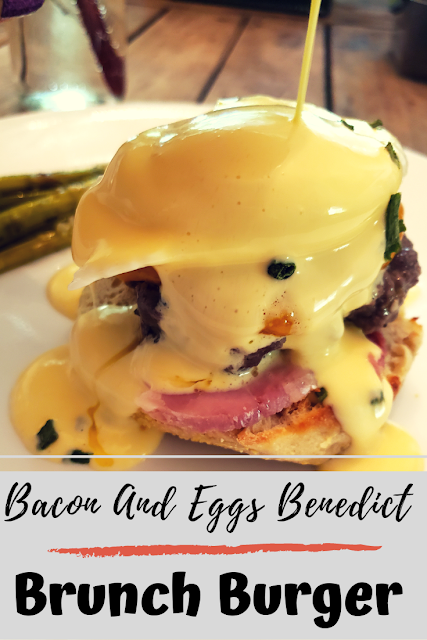This color photograph, presented in portrait orientation, showcases a delectable bacon and eggs Benedict brunch burger prominently centered in the image. The burger is elegantly arranged on a white plate with a brown edge. Atop the burger sits a fried egg lavishly smothered in a creamy, yellow cheese sauce that drips appetizingly down the sides. Beneath the egg, layers of delicious ingredients include a hamburger patty enveloped in more cheese, slices of savory ham, and crispy bacon bits. A hint of green parsley or chives adds a touch of color. A toothpick can be observed sticking out from the upper right corner of the burger, securing its layers. To the left side of the plate, some asparagus or other green vegetables can be glimpsed. The background reveals wooden floors, suggesting the photo was taken inside a restaurant. Beneath the plate, a horizontal rectangle text box in light gray features descriptive text in black script: "Bacon and Eggs Benedict," underscored by a red brushstroke, followed by bold black text stating "Brunch Burger." The image is an example of photographic representationalism in food photography and conveys a mouth-watering meal with rich, intricate details.